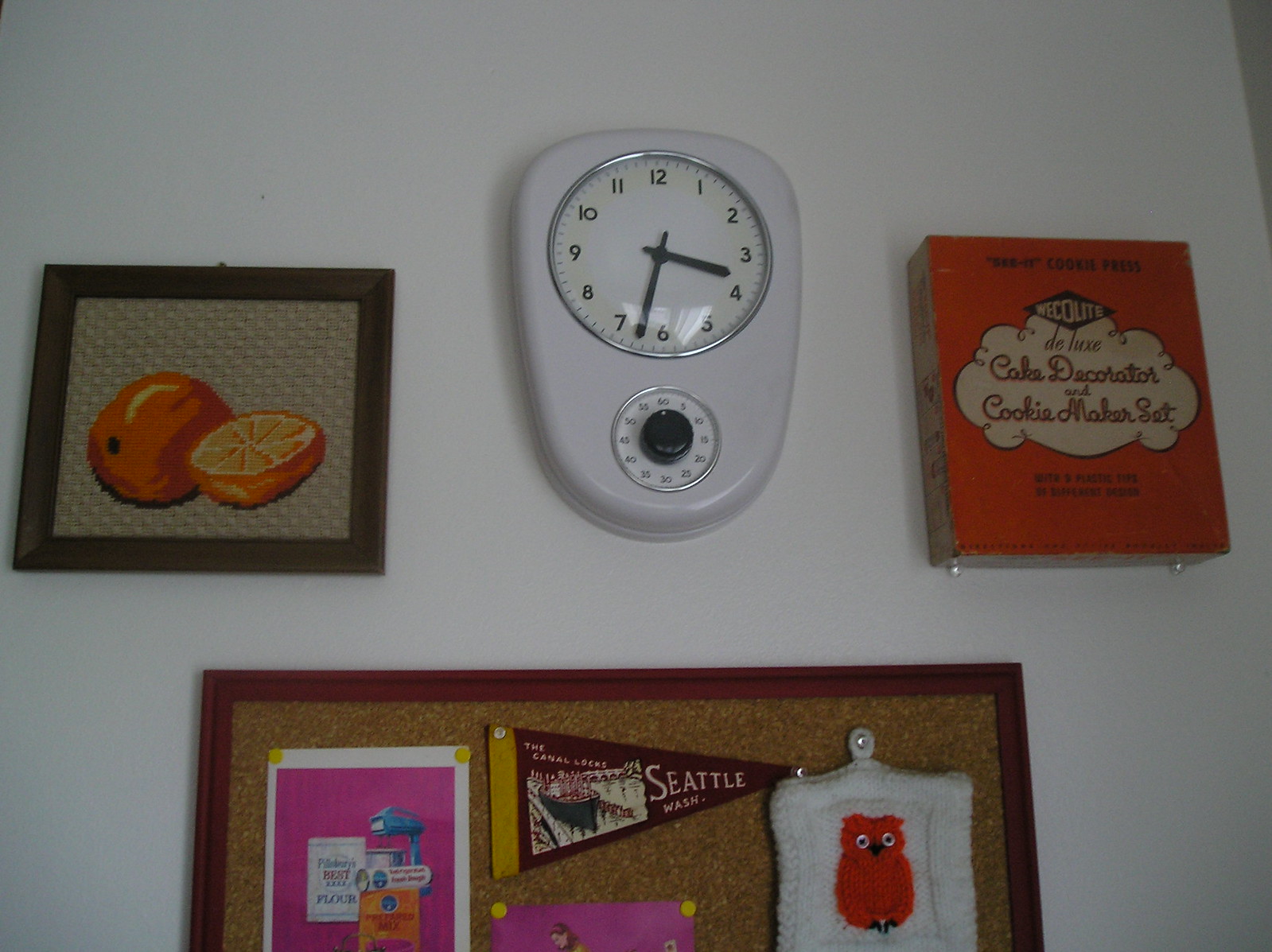The color photograph captures a grey wall adorned with various decorative items, centered around an almost oval-shaped grey clock. The clock features a round face with a silver metallic edge, black numerals, and black hands pointing to approximately 3:35. Below the clock face is a smaller dial with a prominent black button, surrounded by small, unreadable numbers, resembling a weighing scale.

To the left of the clock, there is a framed picture with a dark green edge, depicting an orange fruit on the left and a half-cut orange showing its segments on a beige, textured background. On the right side of the clock, another framed item appears, resembling the cover of a red book. It features a greyish cloud with possibly the word "cola" written on it, followed by some legible joined-up handwriting.

Below these central decorations, a cork board with a dark wooden edge partially comes into view. A dark maroon flag with "Seattle" written in white letters is pinned to the board. Near this flag is a decorated white furry object with a red owl in its center. Adjacent to these items, on the left, there is pink paper with various objects pinned to it. Below the maroon Seattle flag is another smaller pink flag.

The composition creates a complex and visually intriguing wall display, blending functional and decorative elements seamlessly.